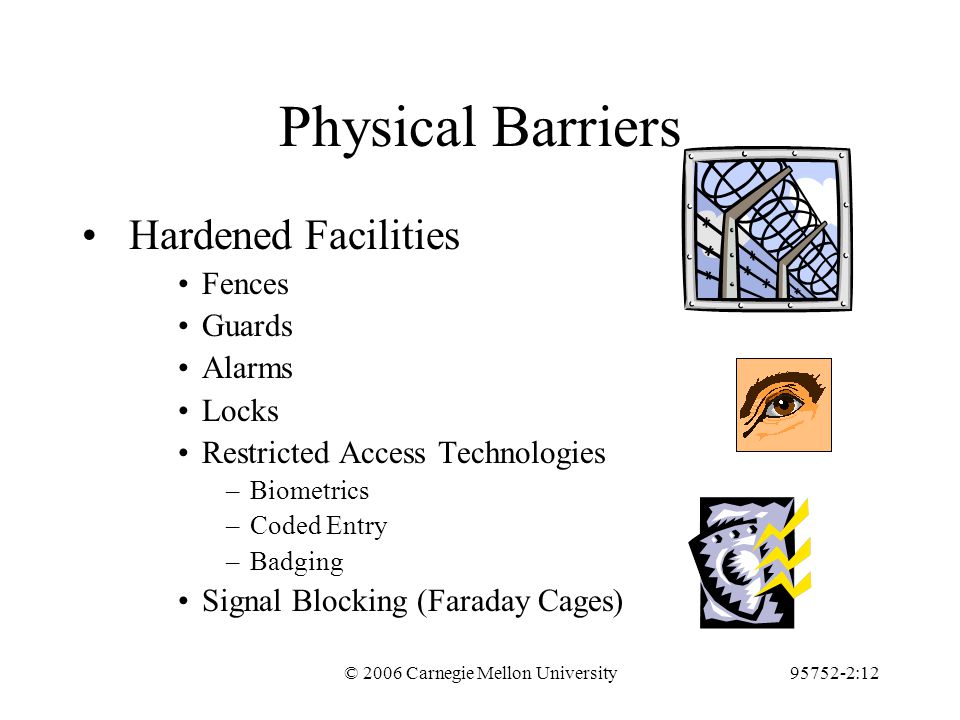The image is an informational slide or card from an educational PowerPoint presentation, featuring a white background with black text predominantly and various pieces of clip art. The main heading at the top reads "Physical Barriers," followed by subheadings such as "Hardened Facilities". Bullet points list terms: "Fences, Guards, Alarms, Locks, Restricted Access Technologies," and below these, there are additional labeled points including "Biometrics, Coded Entry, Badging." Another bullet point reads, "Signal Blocking (Faraday Cages)."

The image includes several colorful clip art pieces positioned to the right side: a picture of barbed wire against blue and white clouds, an eyeball with a brown eyebrow and eyelash, and a shield with yellow lightning bolts striking it. The text at the bottom states, "Copyright 2006, Carnegie Mellon University," and a seemingly random string of numbers and punctuation, "95752-2:12." The colors in the clip art include black, white, blue, gray, orange, brown, light brown, blue-gray, and yellow, lending a varied palette to the otherwise monochrome slide.